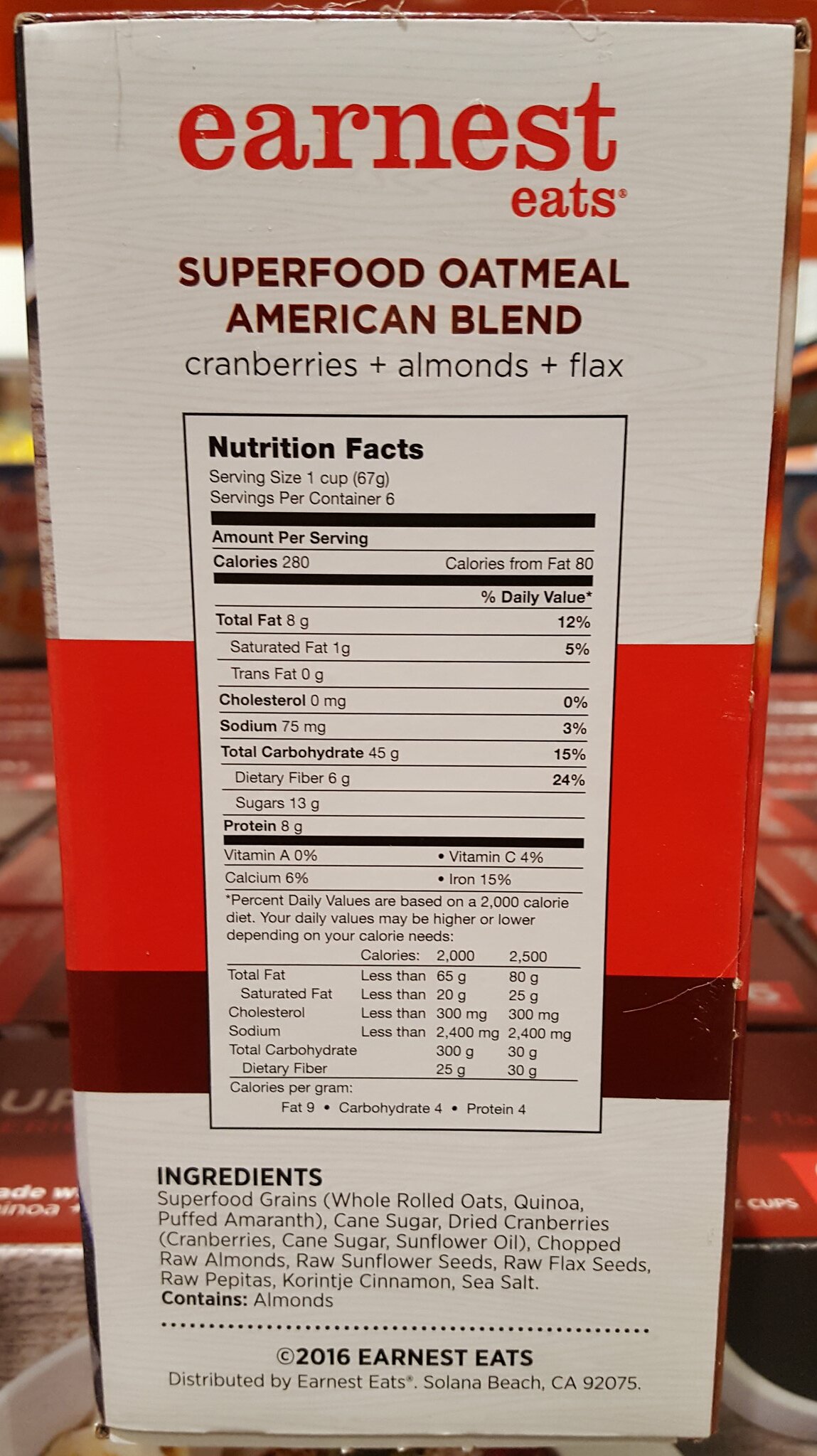This close-up photograph showcases the back of a cardboard oatmeal box, which is taller than it is wide and designed with a clean, minimalist aesthetic. At the top, in lowercase red letters on a white background, it reads "ernest eats." Below that, in maroon text, it says "Superfood Oatmeal American Blend," followed by "Cranberries + Almonds + Flax." Spanning the center of the box is the standard U.S. Nutrition Facts label, which occupies about half the height of the box. The background features a red stripe transitioning into a darker red in the middle section, and a brown stripe at the bottom. Below the Nutrition Facts, there is an ingredients list, also on a white background, followed by copyright information stating, "Copyright 2016, Ernest Eats. Distributed by Ernest Eats, Solana Beach, California, 92075." The box indicates that one serving contains 280 calories.